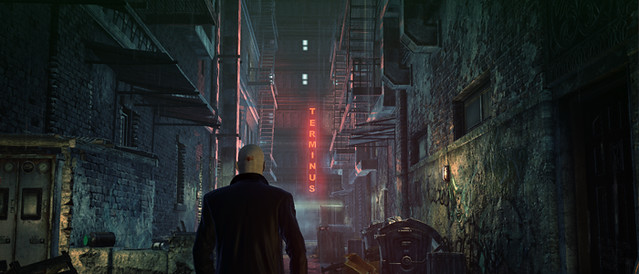The caption describes a still image from the video game "Stock Exchange." In the image, a man walks down a very dark, foreboding alley. The atmosphere is distinctly sinister, evoked by the surrounding shadows and grimy environment. The man, viewed only from the back, wears a black jacket. His identity remains ambiguous, but a peculiar detail—a chip or perhaps an eye embedded in the back of his head—suggests he might be a robot. He is bald, and his skin, difficult to discern in the low light, appears either gray or white, suggesting a Caucasian origin.

To his left, a series of fire escapes are visible, adding to the claustrophobic feel of the narrow alley. A notable feature is a red, neon, vertical sign ahead of him, reading "Terminus." The ground is cluttered with dumpsters, enhancing the seedy and unkempt atmosphere. The right side of the alley mirrors the left, with more fire escapes and another large dumpster aligned with what appears to be shabby apartment buildings. The overall scene is enveloped in darkness, with the red neon sign casting an ominous glow on the alley's grim surroundings.